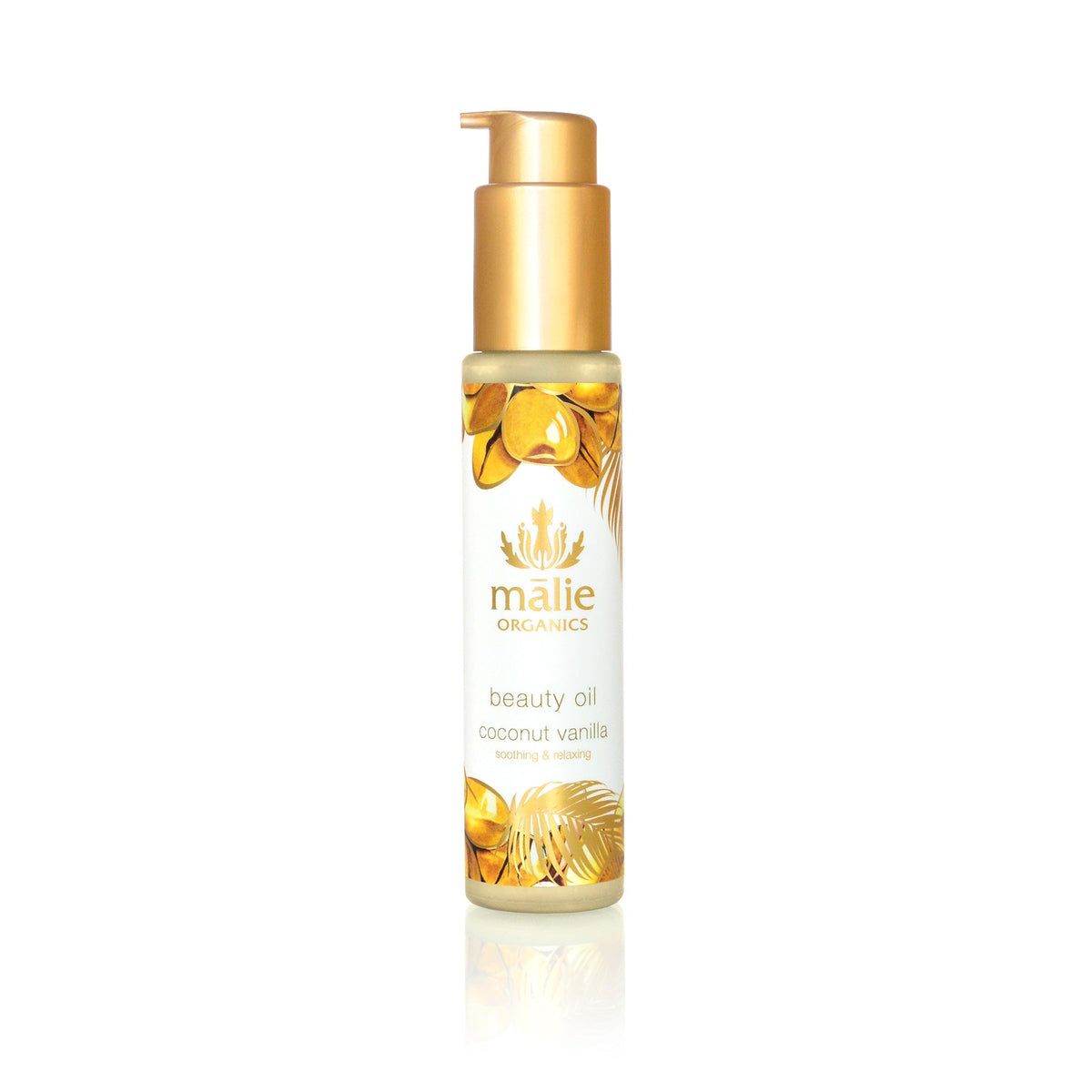This color photograph features a tall, slender canister of Malie Organics Beauty Oil, coconut vanilla. The bottle, approximately eight to nine inches in height with a diameter of a couple of inches, is positioned against a stark white background with a faint reflection beneath it. The bottle itself is made of clear or translucent plastic, predominantly covered by a large white label adorned with gold decorative elements and text. The top of the bottle is a shiny gold pump designed for dispensing the oil. The label includes illustrations of gold leaves and what seems to be vanilla and coconut motifs, with the text "Malie Organics" in gold at the top and "beauty oil, coconut vanilla" in smaller black print. The details on the label also hint at soothing and nurturing properties, although some finer text is too small to decipher.